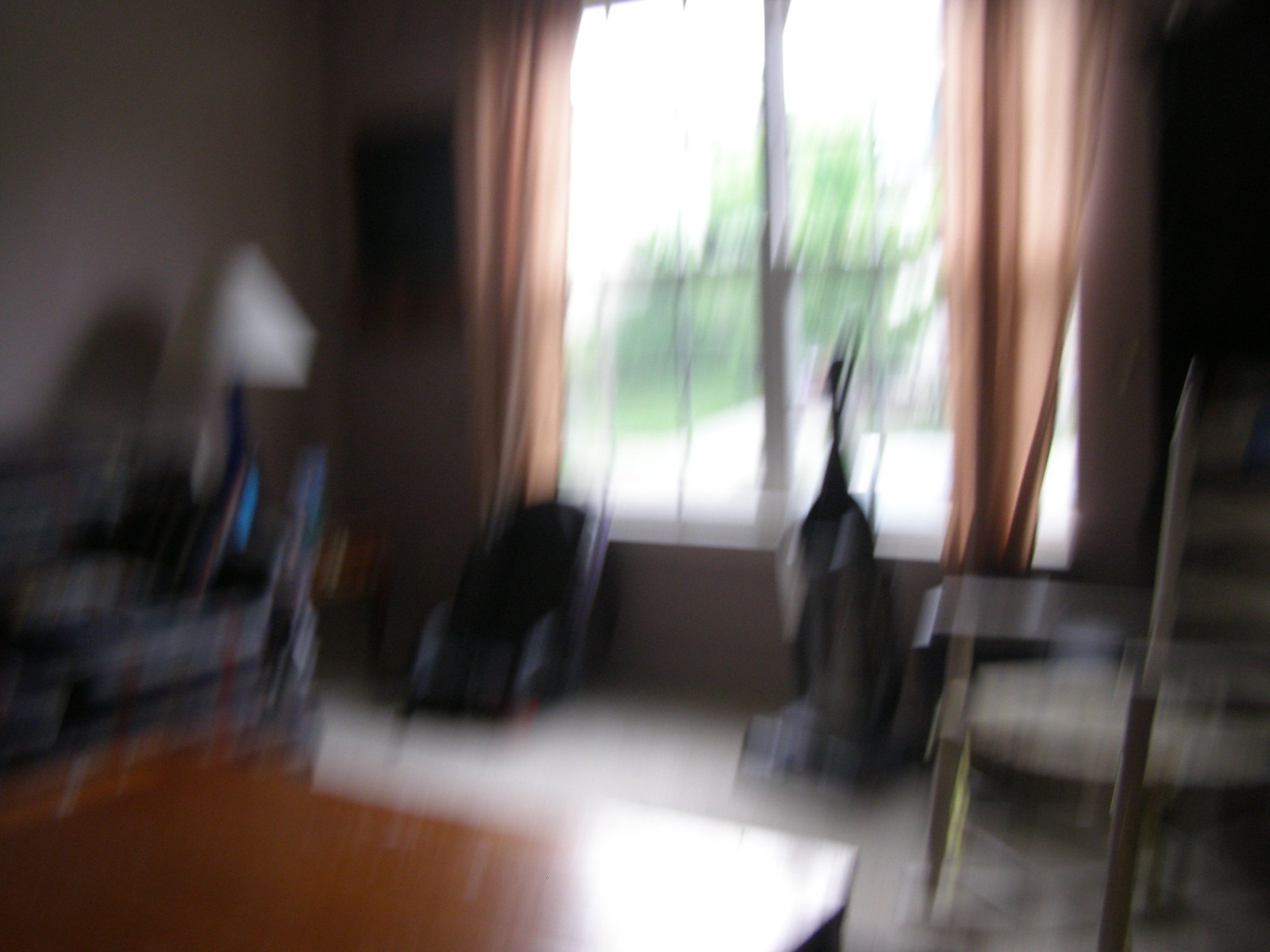This extremely blurry photograph captures the interior of a cozy living room, characterized by a large vertical rectangular window with a cross pane divider, creating four sections. The window, adorned with sheer light beige curtains, allows sunlight to filter through, illuminating the greenery of the trees outside. Below the window, slightly to the right, stands a vacuum cleaner with a rectangular base and an upright stick. On the left side of the window, what appears to be a baby seat is visible on the floor.

In the right portion of the image, there seems to be a glass table, while further right, a wooden chair with a white cushion can be spotted. The foreground showcases a brown wooden coffee table reflecting the incoming light. On the left side of the room, a gray couch is partially in view, adorned with a color print. Next to this couch is a small table supporting a lamp with a blue body and white lampshade. The entire scene is set against a light grayish-white carpet, contributing to the soft ambiance of the space. The image's heavy blurriness suggests it was taken with an unstable hand, resulting in the entire scene being out of focus.